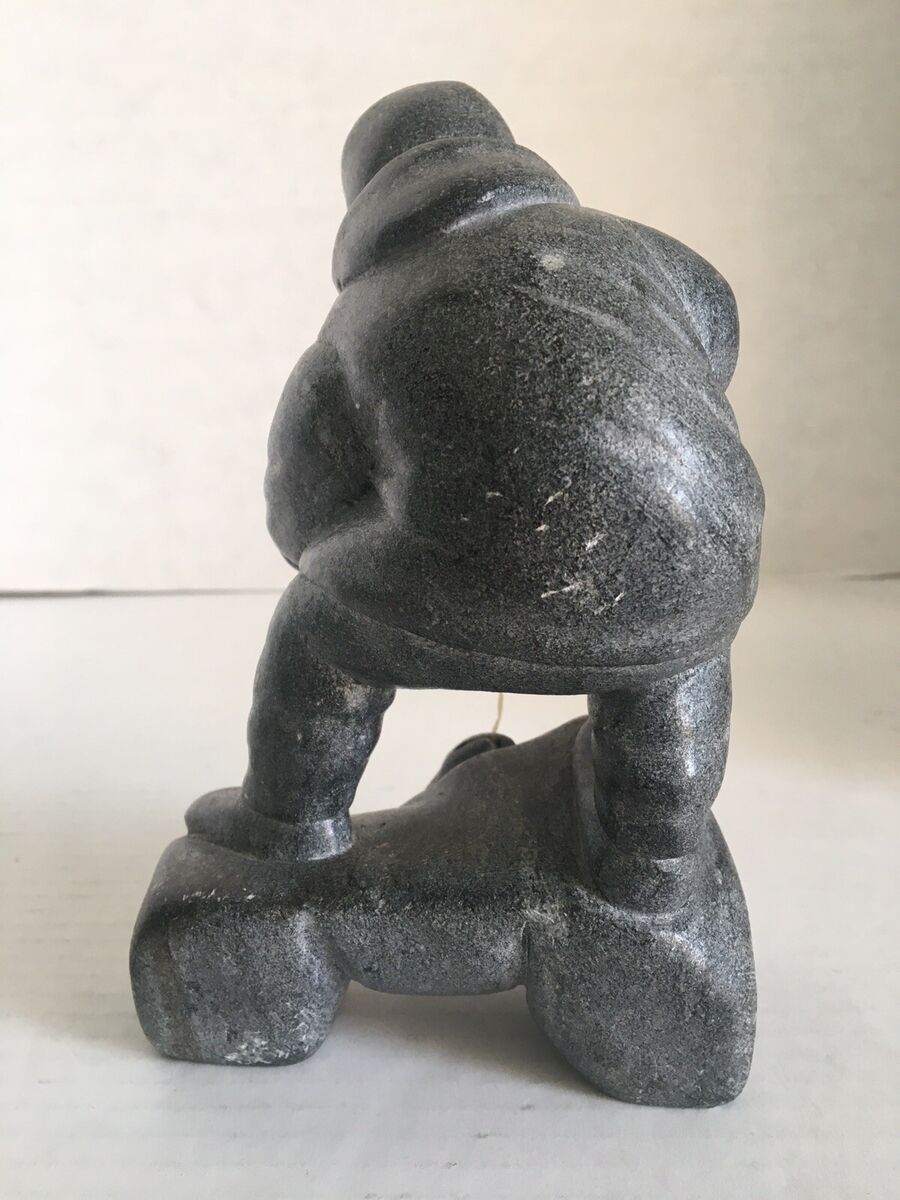In this indoor scene, an old-looking, possibly iron statue stands as the centerpiece. Positioned on a flat white surface against a white wall, this gray to black sculpture features a stocky older man with his back to the viewer. The intricately detailed figure is dressed in boots, pants, a jacket with a scarf-like collar, and a top hat. The man is bent over, with his legs squatted and back arched, giving the impression that he is either attempting to pick something up or is in the act of peeing, as humorously suggested by a stream flowing into a container beneath him. The statue stands on a simple pedestal with two side portions touching the surface, while the middle section is elevated. The entire figure has a slight sheen, enhancing its presence in the stark setting.